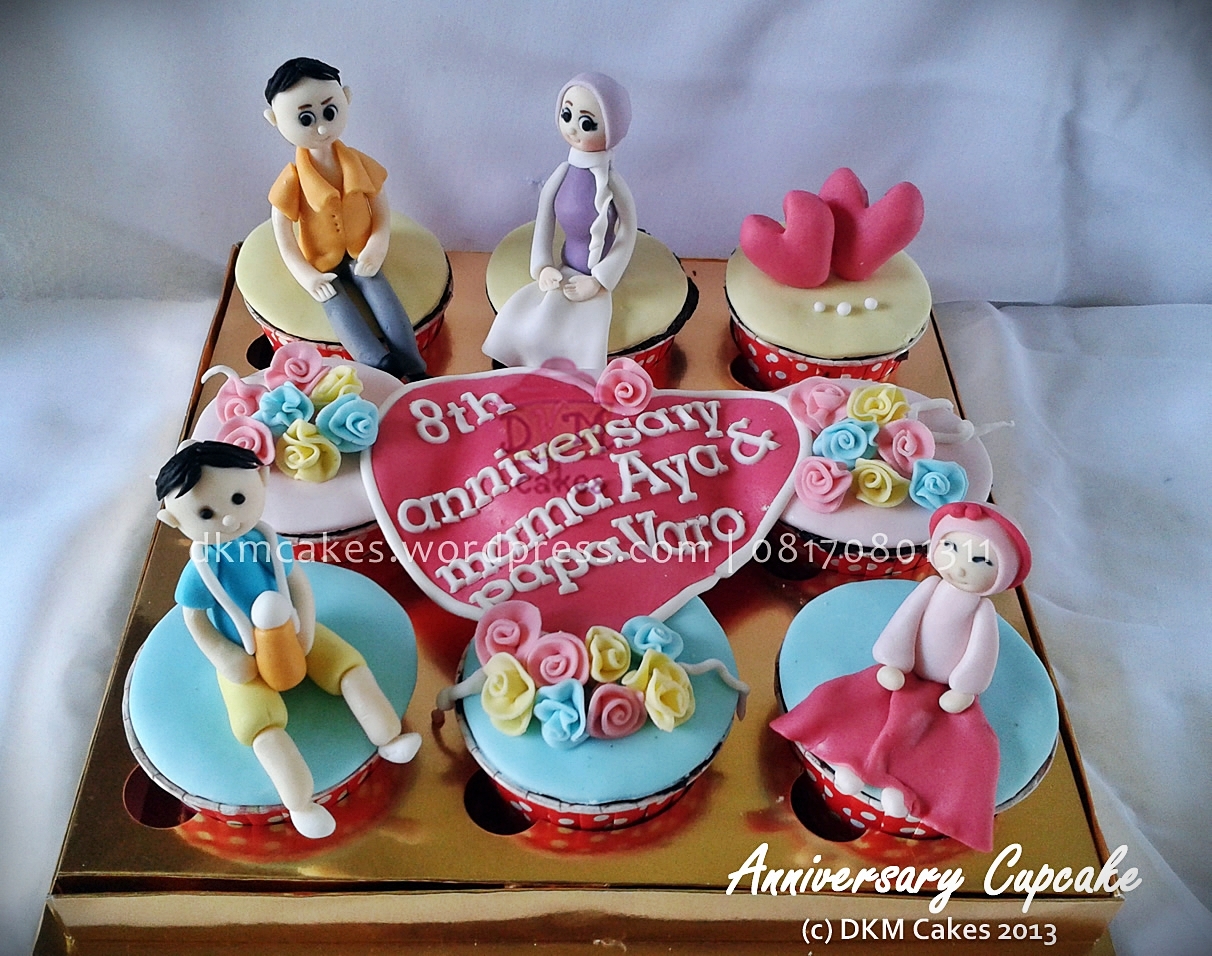This photograph showcases a captivating arrangement of nine custom-decorated cupcakes housed in a gold cardboard box, each nestled in red tins adorned with white spots. Celebrating an 8th Anniversary, a fondant stretches across the cupcakes, reading "8th Anniversary Mama Aya and Papa Varo" prominently in the center. The backdrop is a cloth that also extends underneath the box. Each cupcake features unique decorations: the back row hosts a man and a woman sitting on separate cupcakes, while one in the front displays a little boy holding a drink and another features a girl in a long dress. Three cupcakes are adorned with delicate flowers, one boasts two red hearts, and an additional inscription at the bottom corner reads "Anniversary Cupcake". The bottom right corner of the image is marked with "DKM Cakes 2013," commemorating the creators and the year.